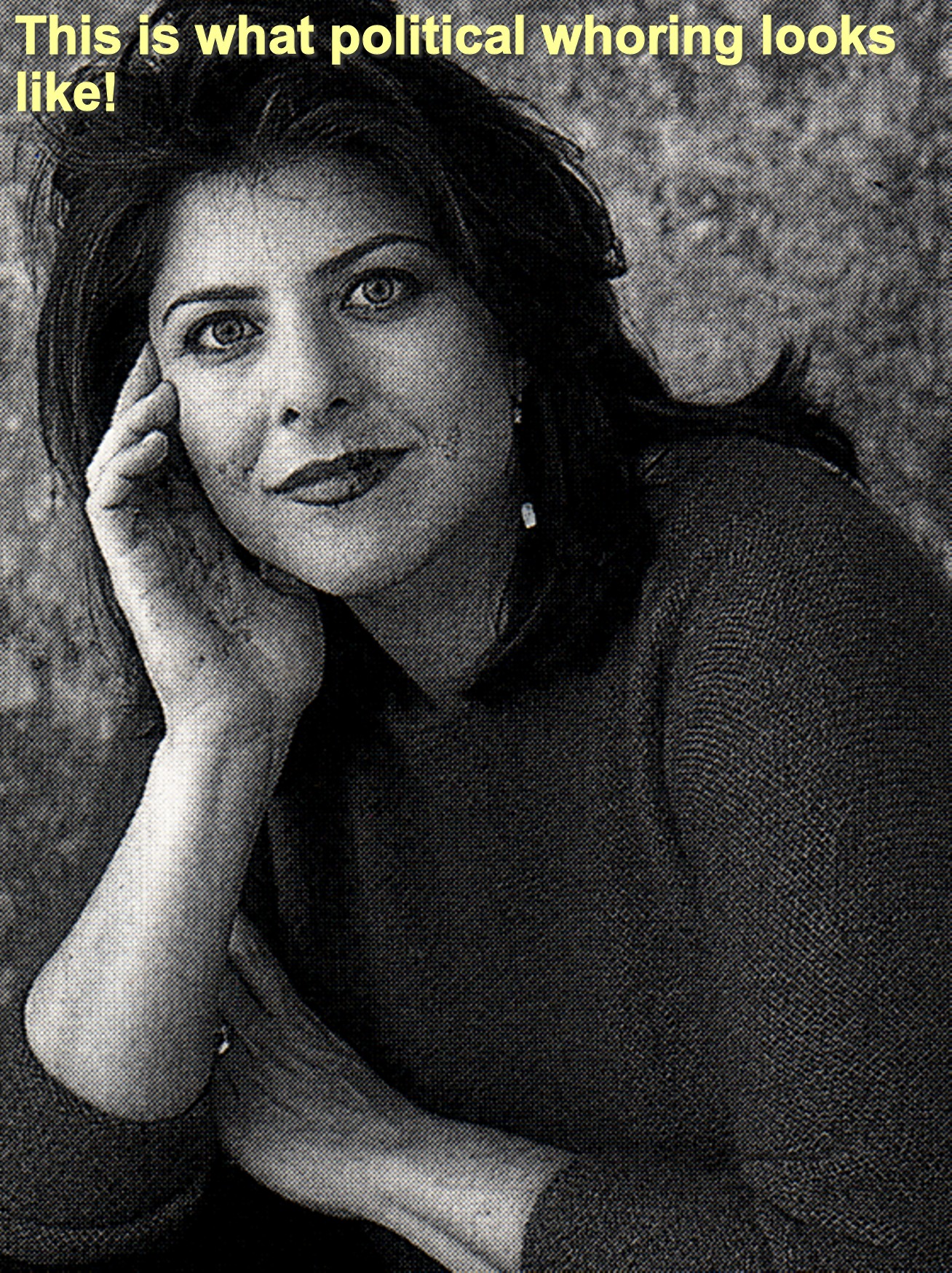This black and white photograph features feminist author Naomi Wolf, known for her influential works including "The Beauty Myth." In this promotional image, Naomi is smiling directly at the camera, with her right cheek resting on her right palm and her left arm crossed in front of her. She wears noticeable makeup, including dark lipstick, eyeliner, and drawn eyebrows. Her dark, medium-length hair falls just past her shoulders. She is dressed in a long-sleeved sweater with rolled-up sleeves, and small earrings can be seen. The background appears to be a marble wall, adding a textured backdrop to the portrait. Added to the top of the image in yellow text is the controversial caption: "This is what political whoring looks like."